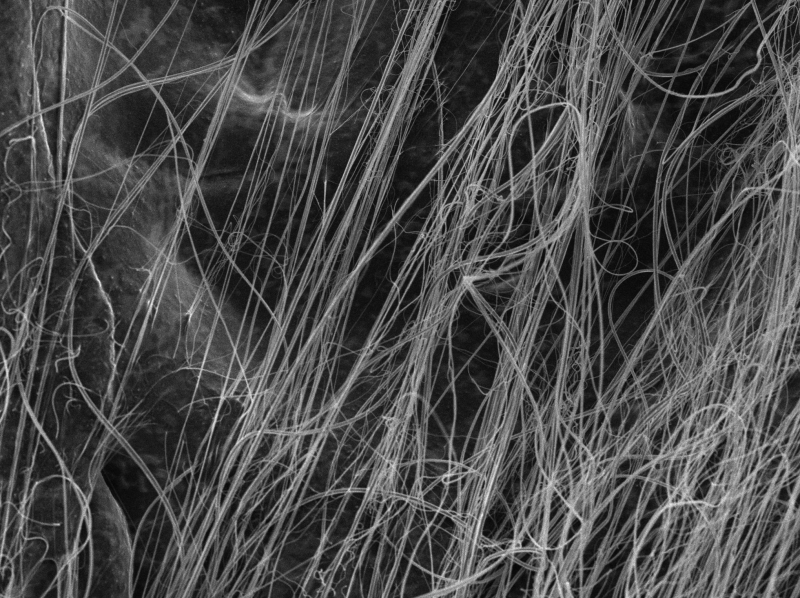This black-and-white image is a detailed, intricate composition of thin white lines set against a starkly contrasting backdrop of dark black and light gray tones. The lines are varied, featuring curved and wispy strokes that resemble dried sawgrass or swirling smoke. These streaks and circles are closely packed, some forming loose spirals and semi-tight curves, while others stretch straight across, creating a layered, almost three-dimensional effect. The overall image is reminiscent of the ghostly trails left by a sparkler, with each white line sharply standing out as if part of an x-ray or photographic negative. The absence of additional elements and the random direction of the lines enhance the ethereal, abstract nature of this artwork.